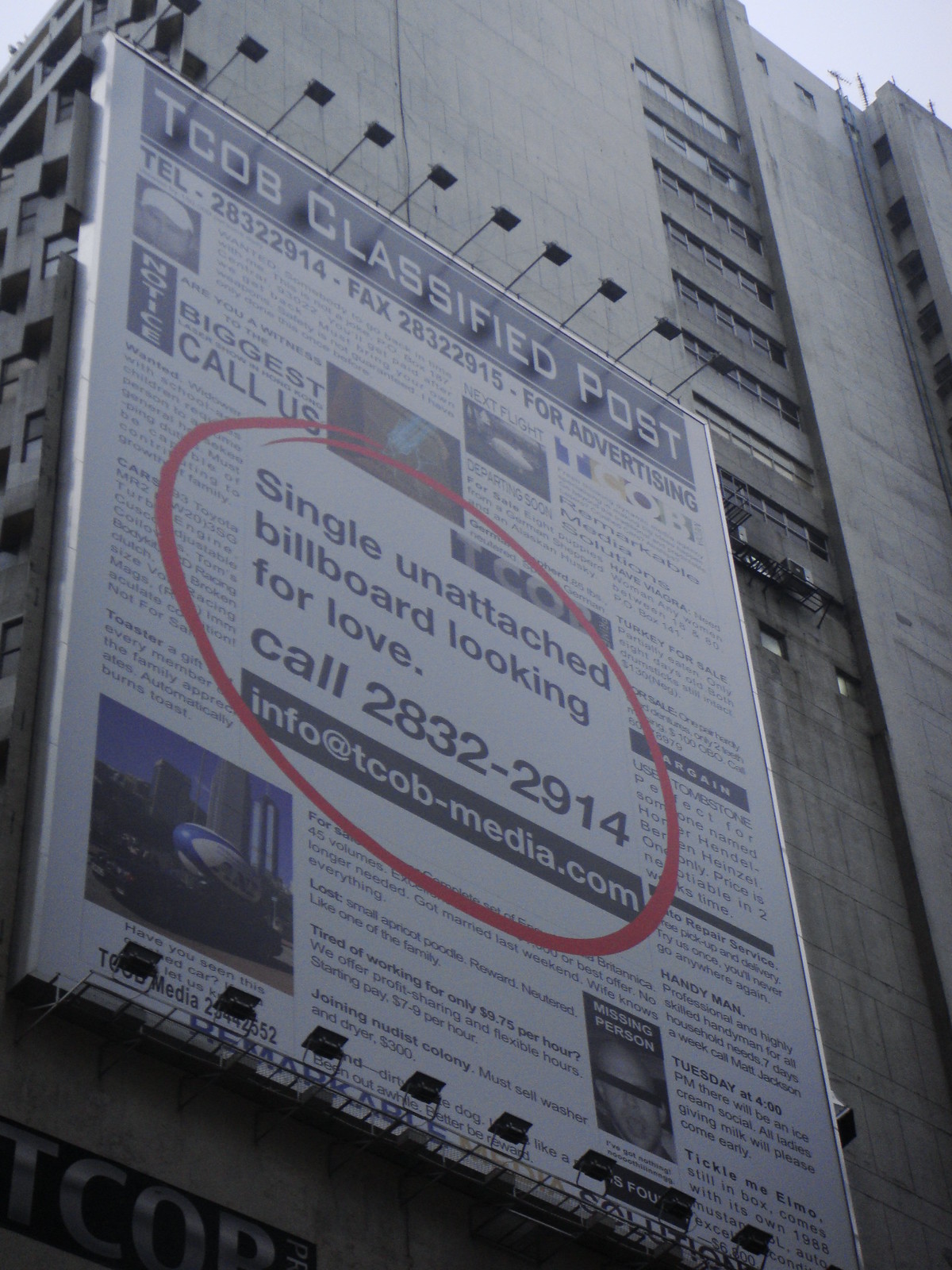The image depicts a large billboard attached to the side of a tall, gray building. The billboard features a prominent navy blue section at the top with white text, while the main area of the billboard is white with black writing. In the center of the billboard, there is an intriguing message that reads, "Single, unattached billboard looking for love. Call [PHONE NUMBER]." A website is also listed: "info@tco-media.com."

The billboard includes other elements such as what appears to be an airplane or balloon, contributing to the whimsical nature of the display. Additionally, there is an image of a man in the lower right-hand corner. The overall design suggests an artistic or unconventional advertising approach, and the contact details indicate it might be part of a campaign by TCO Media. The number listed resembles a classified advertisement rather than a standard telephone number, adding to the mystery and charm of the billboard.